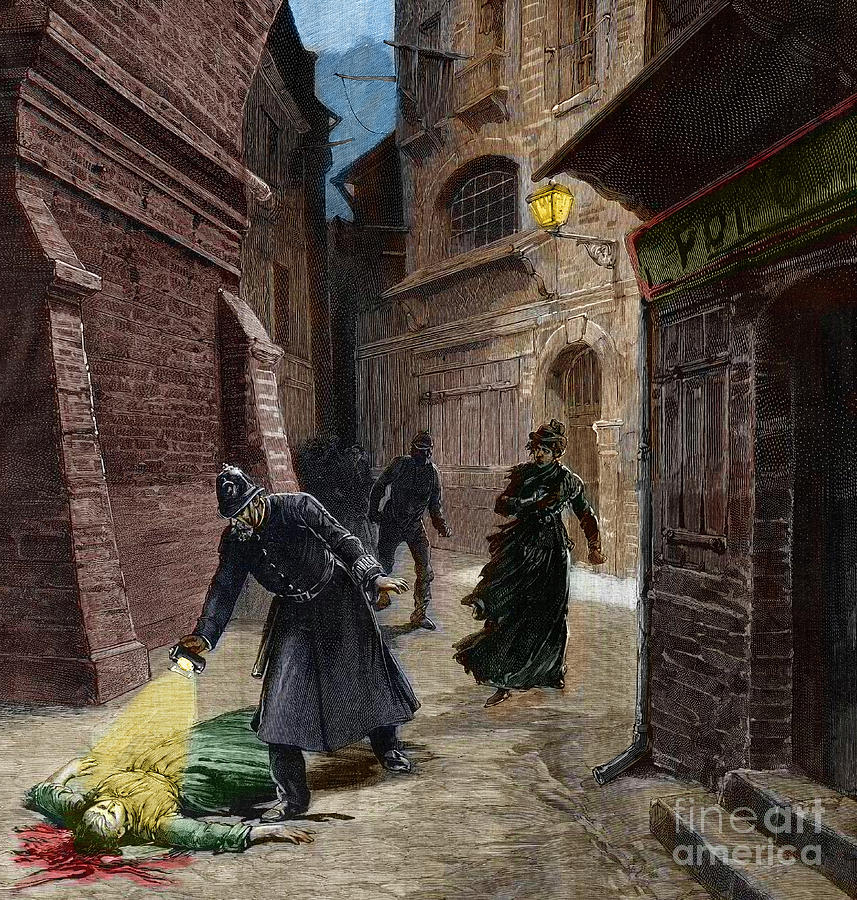The image depicts a grim scene set in a narrow, dark alleyway flanked by tall, old buildings constructed from a mix of stone and rusty brick. Centered in the alley is a police officer in a long black coat and hard hat, crouching slightly and shining a flashlight down on a gravely injured woman lying on the ground. The woman, dressed in a green dress, is surrounded by a pool of blood originating from her head. This tragic tableau is illuminated by a stark beam of yellow light from the officer's flashlight. To the officer's right, a streetlight adds to the dim illumination. In the background stands another woman in a black dress with dark hair piled atop her head, and further behind her, a figure dressed in all black lurks in the shadows. The lower right corner of the image bears the watermark "Fine Art America," indicating its source. The alleyway is enveloped in an ominous atmosphere, with the overbearing buildings and scarce natural light from a barely visible sky and mountain range adding to the scene's overall sense of foreboding.